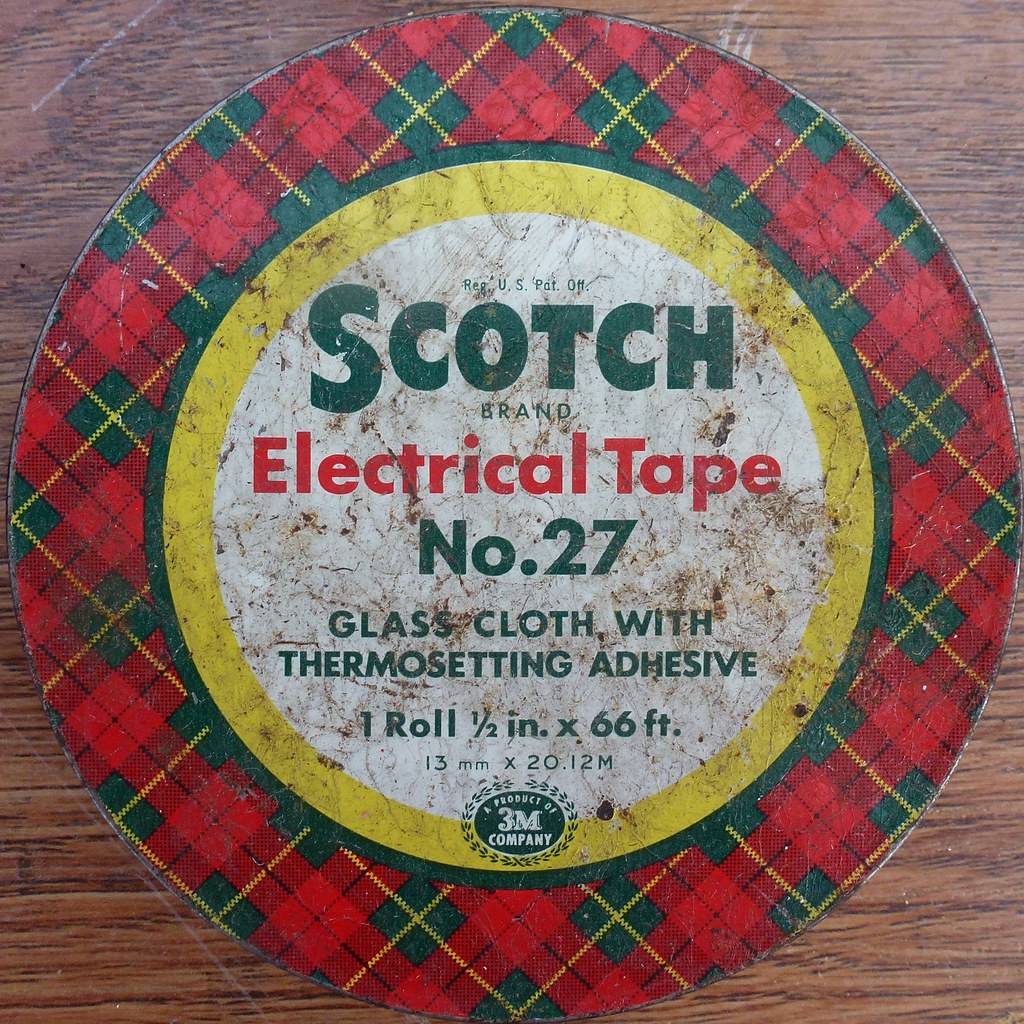The image captures a detailed color photograph of a vintage Scotch brand electrical tape package, specifically No. 27 with thermosetting adhesive. The circular printed cover, prominently positioned in the center of the image, is embedded in a wooden table with a square format. The packaging design features a festive tartan plaid border in red, green, and yellow, with a dark green inner lining and a yellow band framing a white background. In the center, the bold dark green text reads "Scotch" followed by red text for "electrical tape" and "Number 27" in dark green again. Below this, smaller dark green text details the product specifics: "glass, cloth, with thermosetting adhesive," and "one roll, one-half inch by 66 feet." At the bottom, an oval black circle contains the 3M company logo encircled by a black wreath emblem. The vivid colors and meticulous design evoke a sense of nostalgia, capturing the essence of a collectible vintage product in a setting that emphasizes its age and craftsmanship.